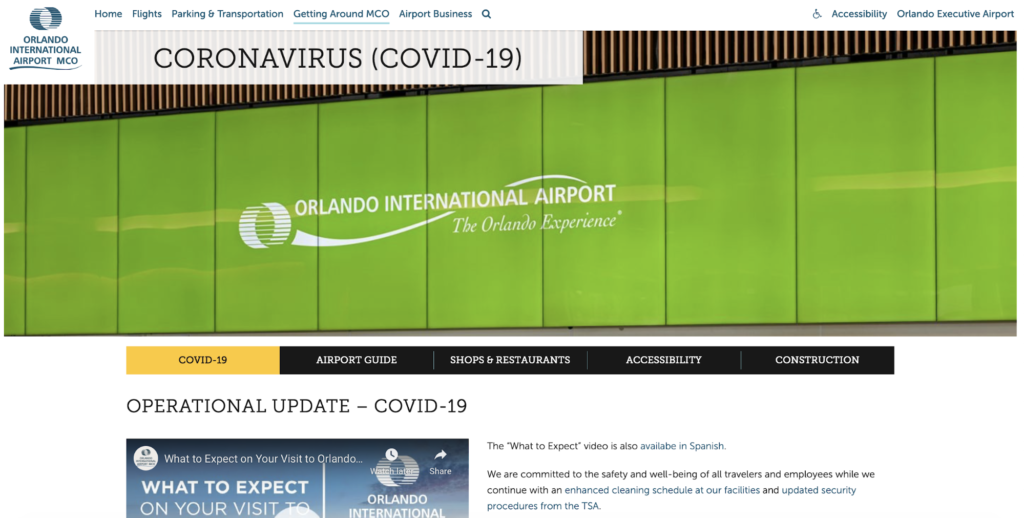The image depicts the official website of Orlando International Airport, prominently displayed in the top left corner. Adjacent to the website name is a highlighted notice about COVID-19, shown in bold yellow text that reads "Coronavirus, COVID-19." The background features a green sign from outside the airport, which proudly states "Orlando International Airport, The Orlando Experience."

Beneath this prominent signage is a navigation bar offering various selections: "COVID-19" highlighted in yellow, while the others are black with white text. The options available are "Airport Guide," "Shop & Restaurants," "Accessibility," and "Construction."

Below the navigation bar is an updated operational notice concerning COVID-19, titled "Operational Update - COVID-19." A small blue box beneath this notice provides further details with the heading "What to Expect on Your Visit to Orlando," displayed on a blue background with white text. To the right, there's a paragraph elaborating on what visitors can expect during their stay at the airport, focusing on the new measures and guidelines implemented during the pandemic.